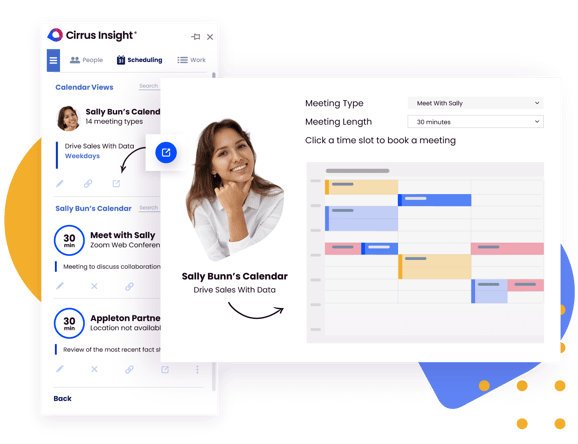This screenshot from a website showcases a user interface heavily utilized by Cirrus Insight. On the left side of the background, there is a prominent mustard yellow circle, and on the right side, a heart-shaped design stands out, characterized by its blue color with scattered mustard-colored dots. Overlapping these background elements, two white pop-up sections provide detailed functionality.

The first pop-up, positioned on the left, is long and narrow, and prominently displays the Cirrus Insight logo along with a pushpin icon and a close (X) button at the top. Beneath these, a blue box houses three lines and various icons – a people icon labeled "people," a calendar icon labeled "scheduling," and a bulleted list icon labeled "work," with the 'scheduling' section currently selected.

Under this selection, headings include "calendar views" and "search." An image of a woman, labeled as Sally Bunn, appears next to text indicating "Sally Bunn's calendar," which is partially cut off. Below this is a list of 14 meeting types, with the first one reading "drive sales with data weekdays." Additional information includes a small white box with a blue circle and a share button, accompanied by a black arrow pointing to the share button. Other calendar entries include “search,” “30 minutes, meet with Sally, Zoom web conference, meeting to discuss collaboration,” and “30 minutes, Appleton partners, location not available, review of the most recent fact,” which is truncated. Each of these entries features small icons underneath – a pencil, an X, an infinity symbol, and a share button. At the very bottom, the word "back" is displayed.

The second white pop-up prominently features a larger circular profile picture of Sally Bunn. Text reads “Sally Bunn's calendar, drive sales with data,” accompanied by a curved arrow pointing to the right. At the top, labels read “meeting type: meet with Sally,” “meeting length: 30 minutes,” and a directive to “click a time slot to book a meeting.” Below this is a gray day planner-style calendar, possibly spanning Monday through Sunday, divided into 30-minute time blocks marked by various colors – orange segments, blue, and pink – although specific times or labels are unreadable. This detailed layout facilitates scheduling and viewing appointments with visual clarity and ease.